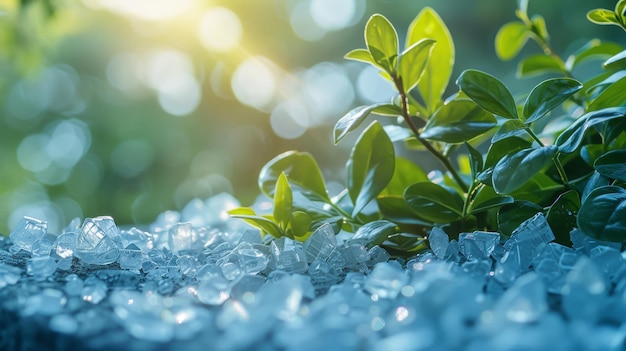This photograph appears to have been taken outdoors and features a multifaceted composition with distinct elements that capture attention at different levels. In the immediate foreground, there are light blue, translucent objects resembling sea glass or bluish crystals. These objects catch and reflect light, creating a shimmering effect and providing an artistic contrast within the image. As you move slightly away from the forefront, the texture and definition of these objects become clearer.

Midway through the picture, primarily extending toward the right side, a variety of foliage is captured in focus. This includes reddish-brown stems intertwined with vibrant green stems, along with small, shiny rounded green leaves. The plant life occupies a substantial portion of the middle to the right sections of the image, increasing in density as it progresses towards the right.

In the upper part of the photograph, the background is blurred, consisting likely of shrubbery or bushes, which provides a soft backdrop that keeps the focus on the foreground elements. The sunlight is prominently present, especially in the upper left corner, where its bright rays cause sunspots and light circles throughout the image, enhancing the ethereal quality of the scene. The overall color palette of the photo combines soothing blues and greens, highlighted by natural sunlight, making it a composition that beautifully blends natural forms and light reflections.